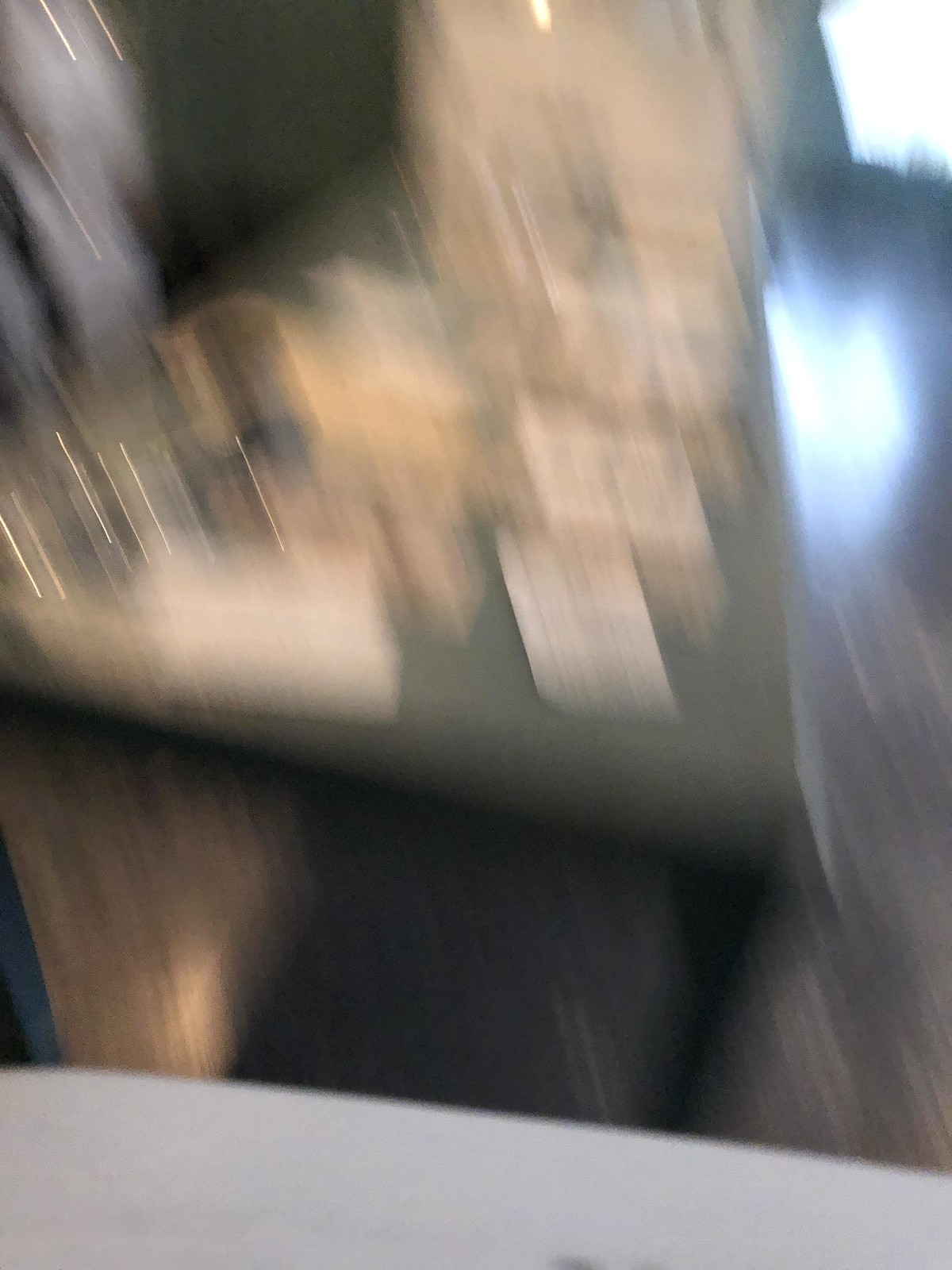This vertical, indoor photograph is characterized by significant motion blur, rendering the scene somewhat indecipherable. At the center of the image is a dark table with black legs and a green tabletop, set against a dark wooden floor. Scattered across the table are various white objects, which could be interpreted as papers, books, napkins, or other light-colored items. These objects appear to reflect light from above, adding to the overall sense of dynamic motion and visual confusion in the photograph.